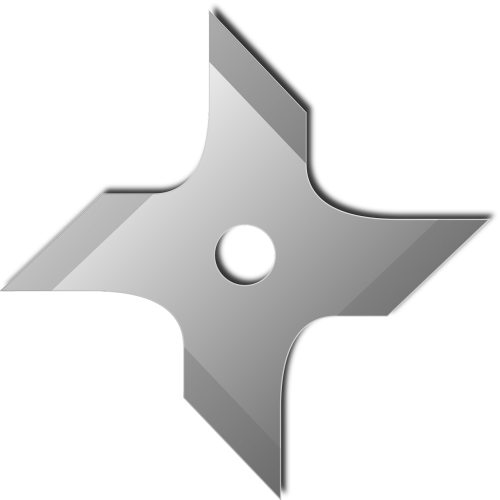The image depicts a silvery-gray, metallic throwing star, also known as a shuriken, set against a plain white background. This implement features a circle cutout at its center, potentially for attaching a handle or improving aerodynamics. The throwing star has four sharply pointed, angled edges oriented in four directions: upward, downward, to the right, and to the left. Each of these edges is darker in color compared to the central section, giving them a razor-like appearance. The points of these edges are angled downward towards a right triangle shape, creating a more sinister and aerodynamic form. The object's edges cast dark shadows, further highlighting their sharpness and curvature. Overall, the design and positioning of the throwing star emphasize its lethal nature and precise craftsmanship.